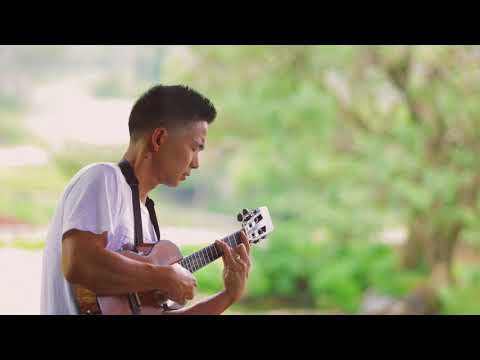In this image, a young man, possibly of Asian descent, is deeply engrossed in playing a small acoustic guitar in an outdoor setting that appears to be a park. He's captured from a side angle, focusing on his concentrated expression and specific hand positions: his left hand is deftly navigating the fretboard while his right hand picks the strings. The man has black hair, tan skin, and is comfortably dressed in a white t-shirt. The harness around his neck secures the guitar, ensuring it remains in place. His subtle grin suggests he is enjoying the moment. The background is blurred but gives hints of a nature-filled environment, with trees and plants, lending a sunny, serene atmosphere to the scene. A strip of black runs horizontally across the image, possibly a bench or fence, further emphasizing the park-like setting.